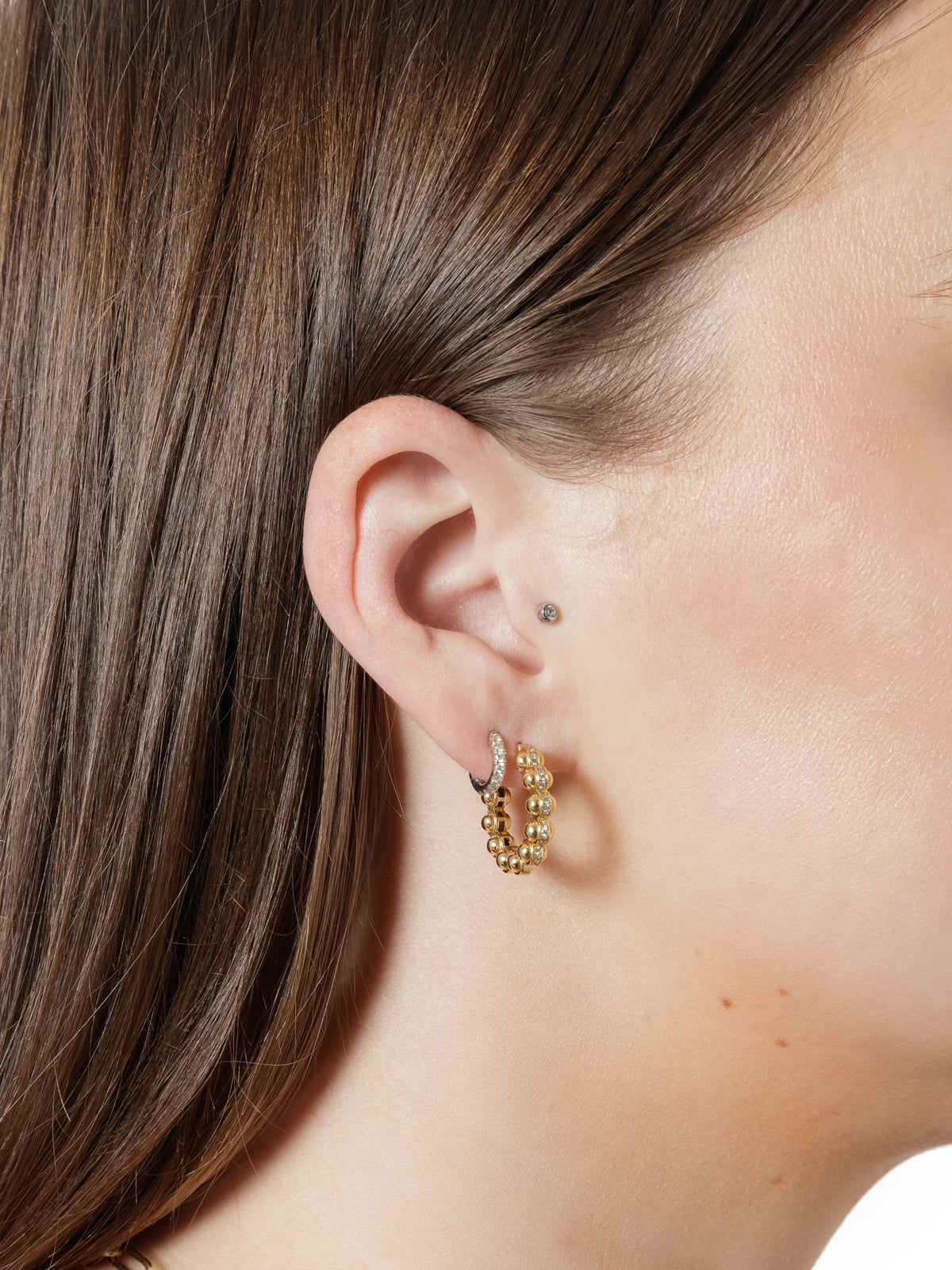This photograph is a close-up of a brunette woman's ear and jawline, showcasing her jewelry. Her straight, neatly tucked hair reveals her small ear adorned with elegant piercings. Her skin is pale and clean, though it features a few beauty spots. Focusing intently on the jewelry, the image highlights three distinct earrings. At the top, a tiny round diamond stud pierces the cartilage. Below, her lobe features two piercings: the forward one is a delicate hoop made of small gold beads, casting a slight shadow on her cheek, and the second is a larger hoop encrusted with small diamonds. The composition, with her ear centrally framed, suggests this close-up is likely part of a product line showcase for jewelry.